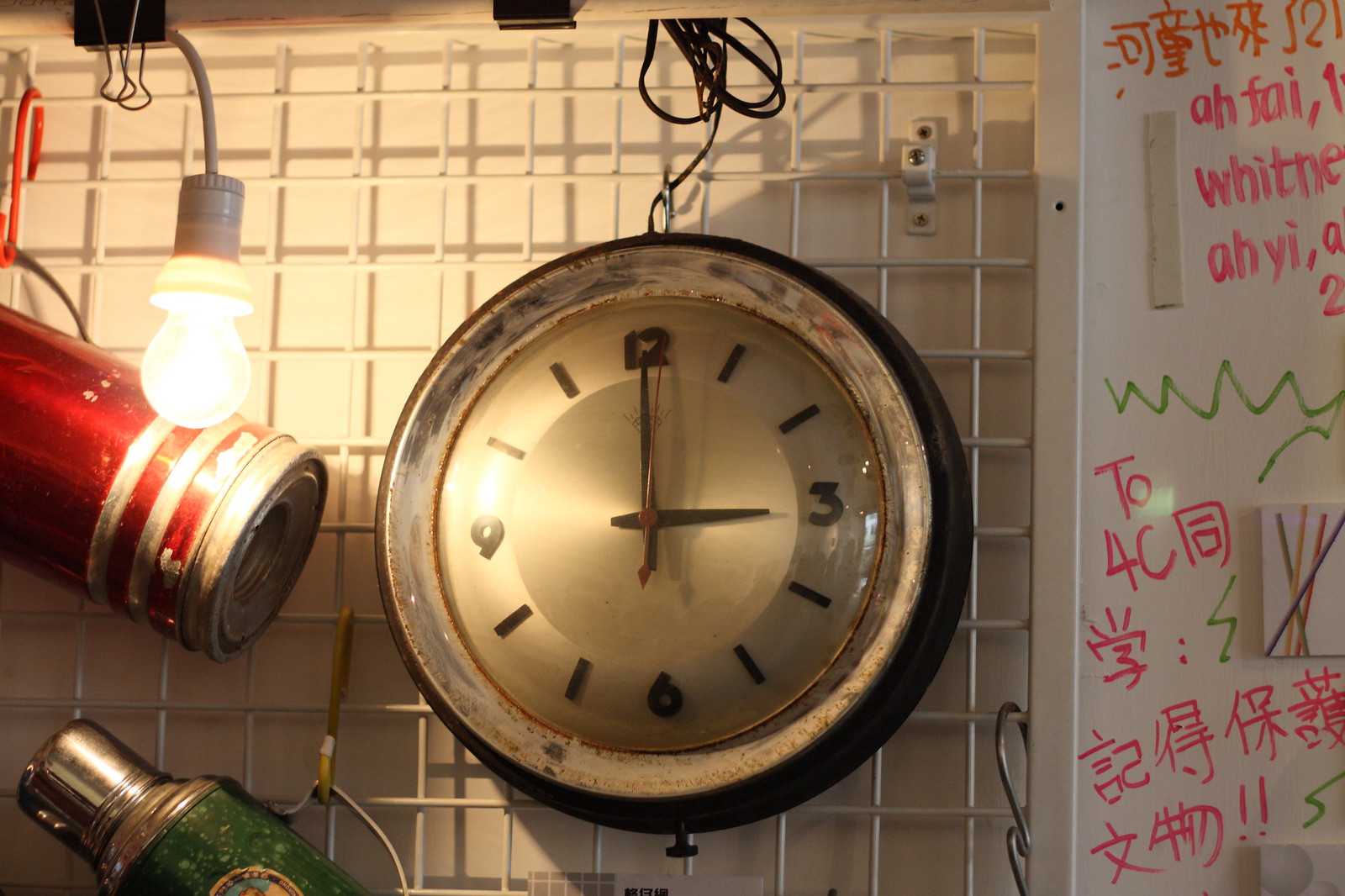The image depicts a detailed storage area scene with a white wire grid frame against a white wall. Centrally hanging on the grid is a large, antique-style wall clock with a brushed silver metallic finish and black hands. The clock features only the numerals 12, 3, 6, and 9, with dashes marking the other hours. It currently reads 3 o'clock. Behind the clock, there is a dark brown disc and visible black wires, though their purpose is unclear. 

To the left of the clock, a bright white light bulb is held up by a black clip with a silver accent. Below the clock, there are two metal thermos bottles: one red and one green, resembling those found in some Asian cultures. On the right side of the grid hangs a whiteboard, partially visible, with handwriting in pink, possibly Chinese characters, and some green zigzag markings. Other words in various languages, such as "Afe," "Whitney," and "Ahi," can also be seen, alongside the pink text "24C." 

Overall, the scene conveys an eclectic mix of objects arranged on a utilitarian wire grid, presenting a blend of functional and cultural elements.